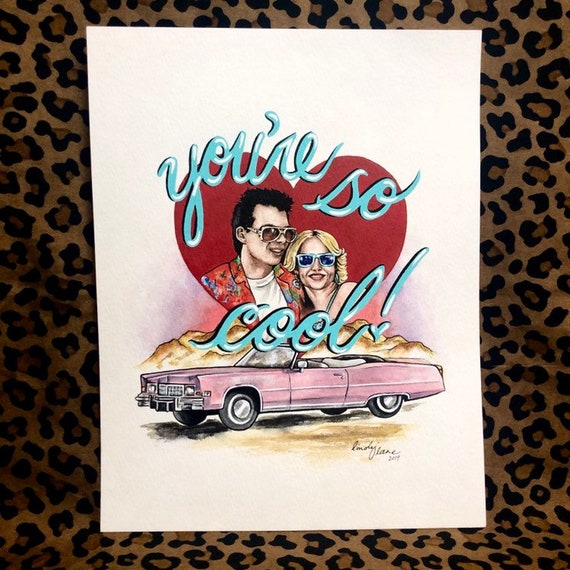The image is an artistic rendering with a vintage tattoo style on white paper, set against a leopard print background. Dominating the top portion of the image is a red heart with blue cursive lettering that reads "You're So Cool!" Inside the heart are a man and woman, both smiling and wearing sunglasses. The man, with spiky black hair, is dressed in a white t-shirt topped with a red, floral-patterned collared shirt, reminiscent of a Hawaiian style. The woman, with 70s styled blonde hair blown back, wears hoop earrings and rests her head on the man’s shoulder. Below the heart, a pink convertible, possibly a Cadillac, cruises in front of a yellow desertscape with brown mountains in the distance. The artist has signed the piece near the rear driver's side wheel of the car.